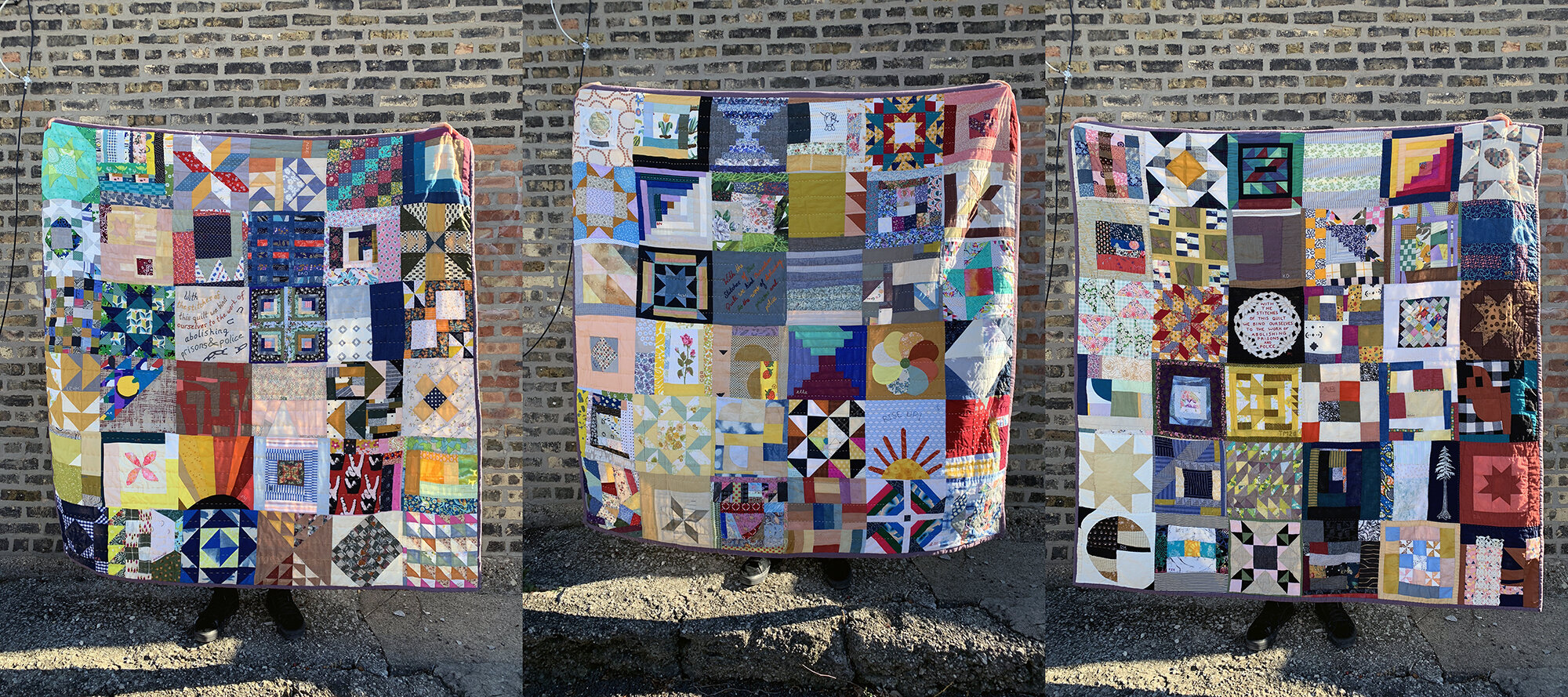The image is a horizontal rectangular collage of three side-by-side photographs, each featuring a person holding up a distinct patchwork quilt. The background of all three photos is a predominantly gray brick building with occasional red brick patterns, adding a touch of color contrast. At the bottom of each photo, the feet of the individuals holding the quilts are visible, clad in black shoes and standing on a dark gray tar or dirt surface.

Each quilt is a square, composed of a 6x6 grid of smaller squares, showcasing diverse patchwork designs. The patterns vary across the quilts, featuring elements such as circles, stars, dots, flags, and flowers. The vibrant color palette includes shades of white, red, blue, pink, orange, brown, black, and green. Although the quilts share some of the same colors, each one is unique with its own artistic flair. There is no text in any part of the image, and the focus remains solely on the craftsmanship of the quilts.